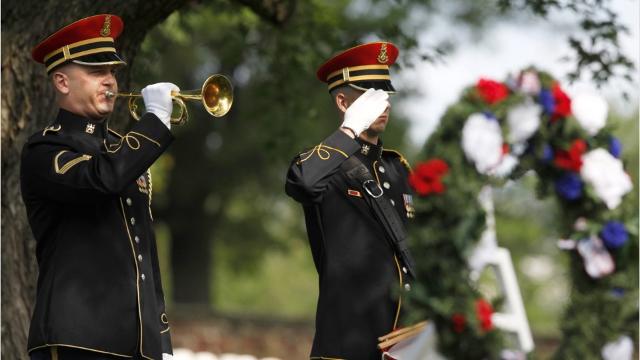In a wide horizontal daytime image, two white male soldiers are captured at what appears to be a cemetery. The sky and green trees blur into the background, but a monumental wreath, adorned with red, white, and blue flowers, stands prominently in the scene, forming a person-sized arch. Closest to the camera, one soldier, dressed in a black uniform with gold buttons, sleeve accents, and a collar emblem, wears white gloves and a black, red, and gold hat with an emblem. He is playing a golden trumpet, holding it with his right hand. Beside him, another soldier, similarly dressed, stands saluting with his hand raised to his hat.